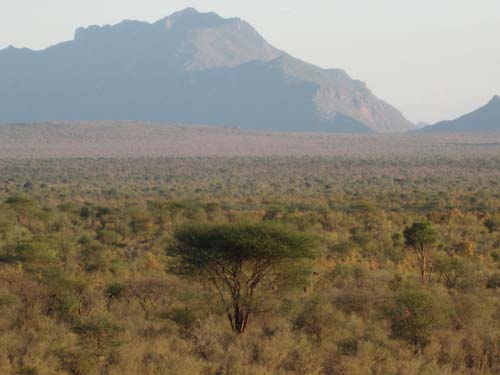This daytime photograph captures an expansive outdoor landscape marked by a serene open plain adorned with low-lying bushes and a patchwork of brown and lightly tan-colored grass. Dominating the background, a strikingly jagged mountain range stretches from the far left, peaks centrally, and gently slopes down towards the right, where a second range begins to fade out of frame. The mountain, hued in dark black or blue, creates a dramatic backdrop against the sky, which shifts between a white and blue gradient.

In the foreground, a solitary tree stands prominently at the center, characterized by its multi-trunked base and a dense canopy of dark green leaves. Further to the right, another smaller tree with a singular stalk and sparser greenery draws attention to the varying flora. The scene is completed with a sprinkling of additional trees and brush, suggesting a rugged, yet beautiful, merger of the greener vegetation with the drier elements of the terrain.